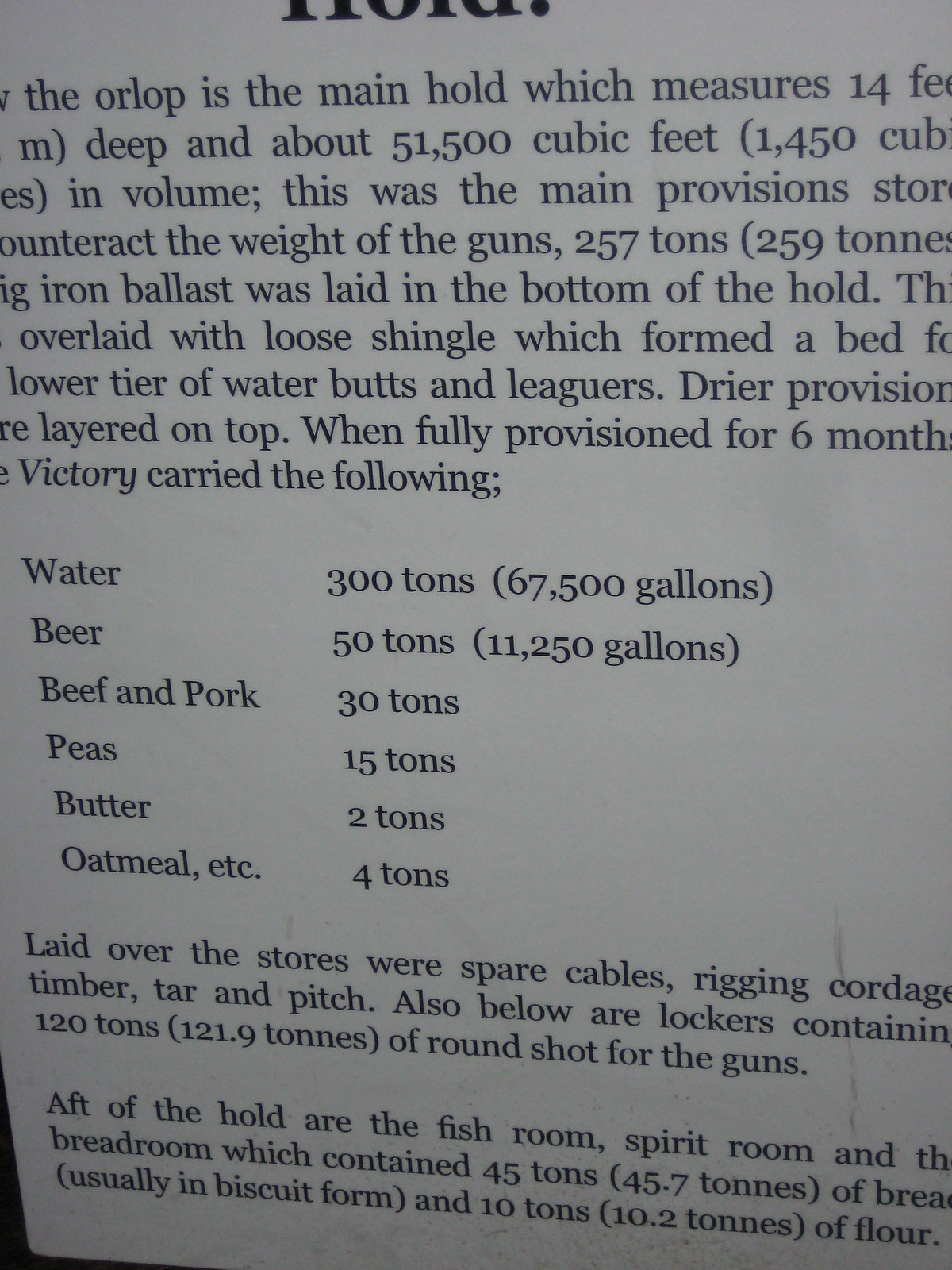The image depicts black text on a dull, grayish-white background with significant portions cut off on the left, right, and especially the top. It describes provisions and accommodations of a ship's Orlop, the main hold, which measures 14 feet deep and about 51,500 cubic feet in volume. The text details that this hold was used for storing provisions to counterbalance the 257 tons of guns. At the bottom of the hold, 257 tons of iron ballast were laid, overlaid with loose shingle to form a bed. The lower tier housed water butts and leaguers with dry provisions layered on top. The ship, when fully provisioned for six months, carried 300 tons of water (67,500 gallons), 50 tons of beer (11,250 gallons), 30 tons of beef and pork, 15 tons of peas, 2 tons of butter, and 4 tons of oatmeal. Additionally, spare cables, rigging, cordage, timber, tar, and pitch were stored above the provisions, and lockers contained 120 tons of round shot for the guns. Aft of the hold were the fish room, spirit room, and bread room, containing 45 tons of biscuit-form bread and 20 tons of flour. At the bottom left of the image, a black area marks the end of the paper.